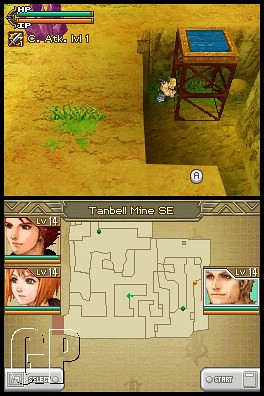This image is a composite from a video game, showcasing two merged screenshots. In the primary image, a towering structure with a flat blue surface dominates the scene, with a character positioned at its base. The surrounding landscape features a mix of brown and green tones, with a grassy patch in the foreground. The upper left corner of the screen displays two status bars: an orange one indicating HP and a blue one for TP. A purple-hued cave is visible in the background, labeled "Tanbell Mine SC."

The secondary element of the composite features a detailed blueprint-style map of the Tanbell Mine, rendered in tan. Three characters are depicted here, presumably the player's current party. Interface elements include a 'Start' button located in the lower right corner and a 'Select' button in the lower left corner, providing navigation options for the player.